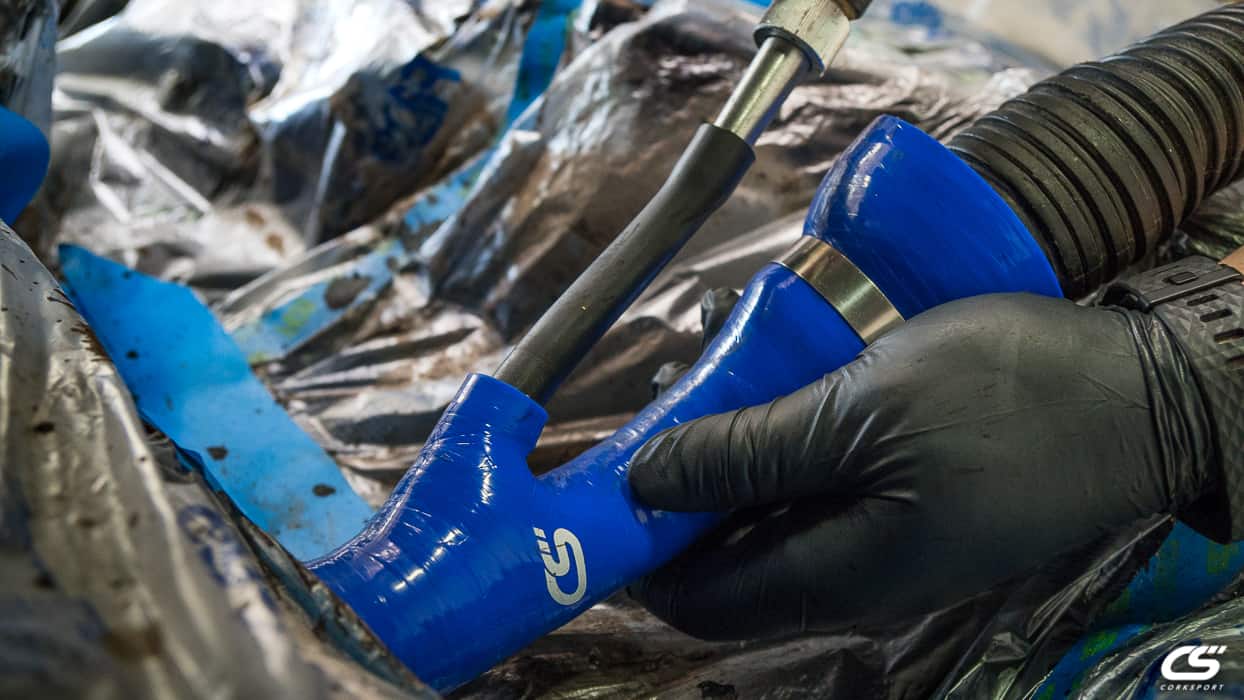A person, possibly working in a technical or maintenance role, is engaged with machinery that appears greasy and covered largely by protective plastic. Blue tape is visible across the machinery, some of it stained with oily or greasy dirt. The worker's left hand, wearing a thick protective glove likely designed for handling hazardous materials, is holding a somewhat plasticky hose resembling those used for water drainage. This hose connects to a vinyl piece that forms a V shape at the bottom and then attaches to a black rubber hose, which in turn is connected to a silver component. Despite the detailed setup, the exact nature of the task remains unclear, though it evidently involves managing some form of fluid, whether liquid or air. A small section of the worker's wrist, where the glove doesn’t cover, is visible, indicating the protective measures taken to prevent contact with potentially harmful substances.